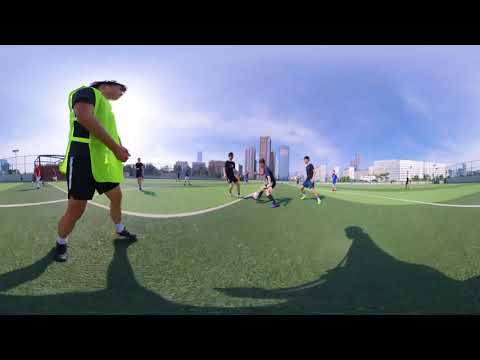In this outdoor photograph taken on a sunny day, a man walks across a grassy soccer field towards the right. He stands out in the foreground wearing a bright fluorescent yellow tunic-style vest that extends down to his legs over a black t-shirt and black shorts. His white socks and black athletic shoes are visible, and he has short, dark hair. His shadow stretches prominently in front of him due to the early or late time of the day, suggested by the long shadows on the field. The lines on the field are slightly curved.

In the background, several young men or teenagers are actively playing soccer. They too are dressed in black shorts and black t-shirts, engrossed in their game amid the warm weather. The sky above is a clear, bright blue with a few scattered clouds.

Beyond the field, the horizon showcases an urban landscape featuring an array of tall buildings, forming what appears to be a city skyline. Notably, there is a large white building to the right. This bustling urban setting provides a stark contrast to the athletic activity in the foreground.